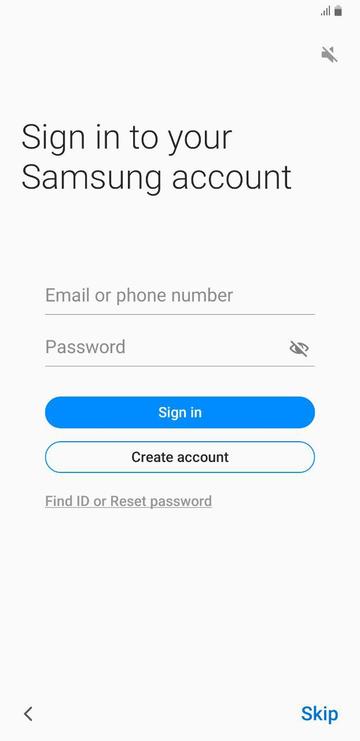In the image, we see a sign-in screen for a mobile app, likely on a Samsung device. The top right corner displays several icons: a battery icon, a Wi-Fi icon, and a sound icon with a line through it, indicating the sound is off. These icons are rendered in a dark gray or nearly black color. 

On the left side, there is prominent black text that reads "Sign into your Samsung account." Below, there are two input fields; the first, with gray placeholder text, prompts users to enter their "Email or phone number," and features an underline. The second field is for the password, marked by the placeholder text "Password" and an eye icon with a slash through it on the far right side, indicating that the password typed will be obscured for security.

Below the input fields, there are two distinct buttons: a blue button with white text that says "Sign In" and a white button with black text that says "Create Account." Underneath the "Create Account" button, aligned to the left, is a link that reads "Find ID or Reset password."

At the bottom of the screen, on the far left, there's a left-pointing arrow, resembling a less-than sign ("<"), likely meant to navigate back to the previous page. On the lower right, there is a link with blue text that reads "Skip," offering an alternative navigation option.